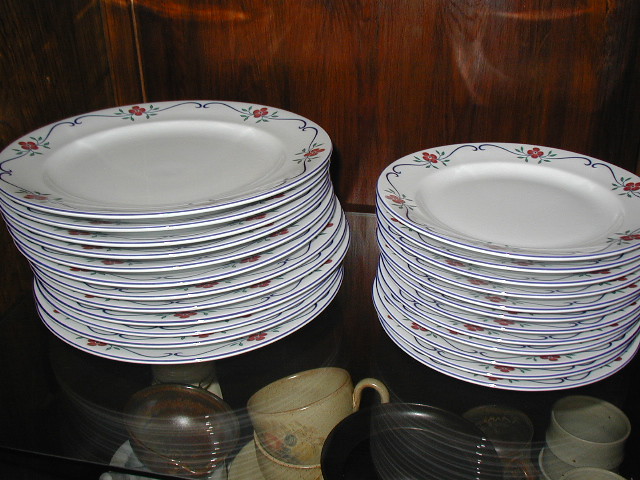The image depicts two uneven stacks of white plates arranged on a glass shelf, set against a dark reddish or dark brown wooden background. The left stack, which is taller, consists of larger dinner plates, while the right stack features slightly smaller salad plates. Each plate sports a Scandinavian or Dutch-inspired design, characterized by a navy blue stripe along the edge and a motif of red flowers with black vines encircling the rim. Below the glass shelf, there is an assortment of serving ware, including ornate teacups, beige coffee cups with floral designs, a black plate standing on its side, and various coffee mugs. The intricate setup is clearly visible thanks to the transparency of the glass shelf.